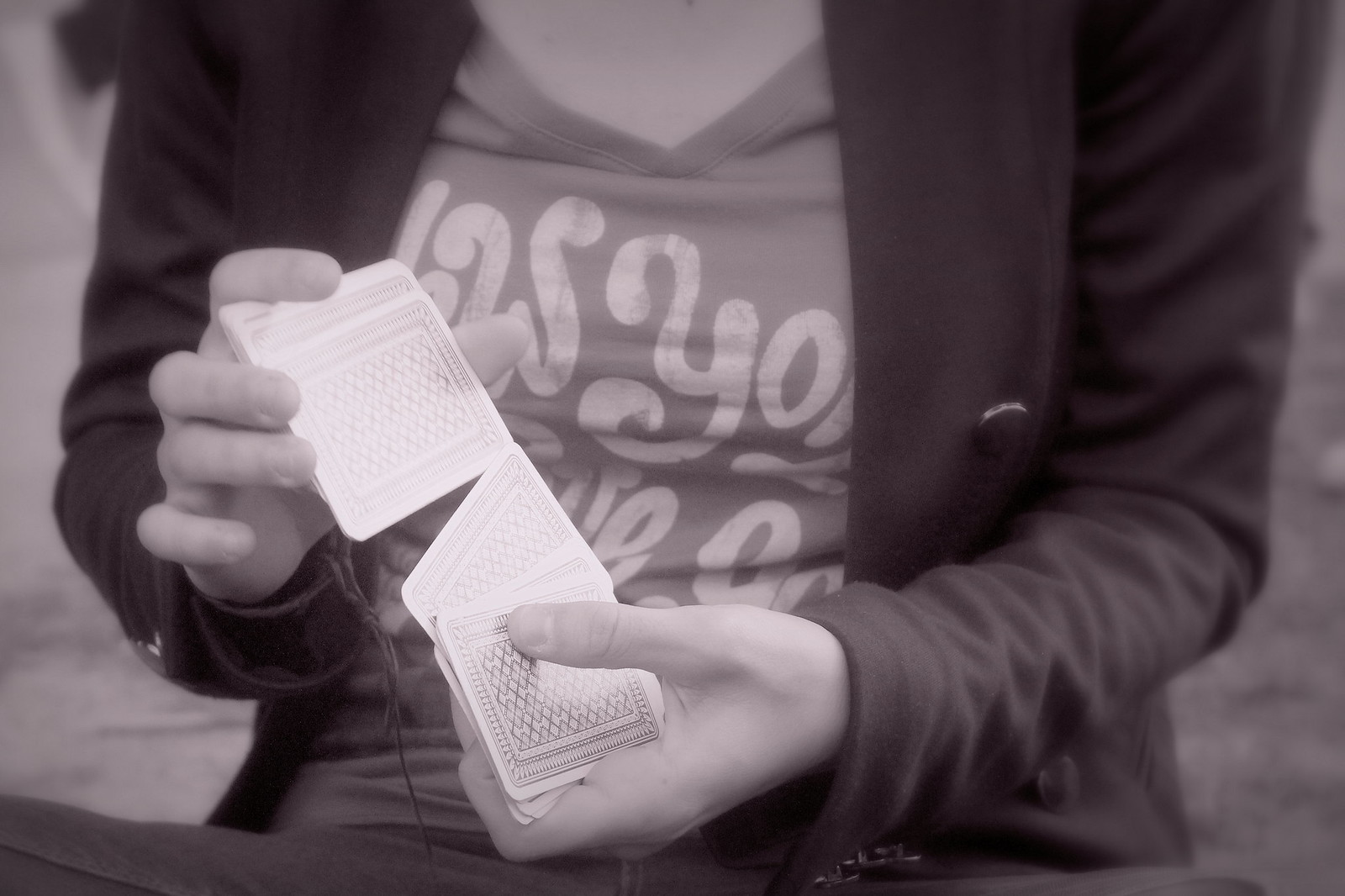The black and white photograph offers an intimate close-up of a woman, captured from below her neck down to her torso. She is dressed in a v-necked t-shirt partially obscured by a dark-colored jacket. Although there are words printed on the t-shirt, they are unreadable as her hands are raised in front of her, actively shuffling a deck of cards from one hand to the other. The intricate back design of the cards is visible, but the particular cards remain unknown. Her outfit is completed with a pair of denim pants, creating a casual yet focused atmosphere as she engages in the card shuffle.